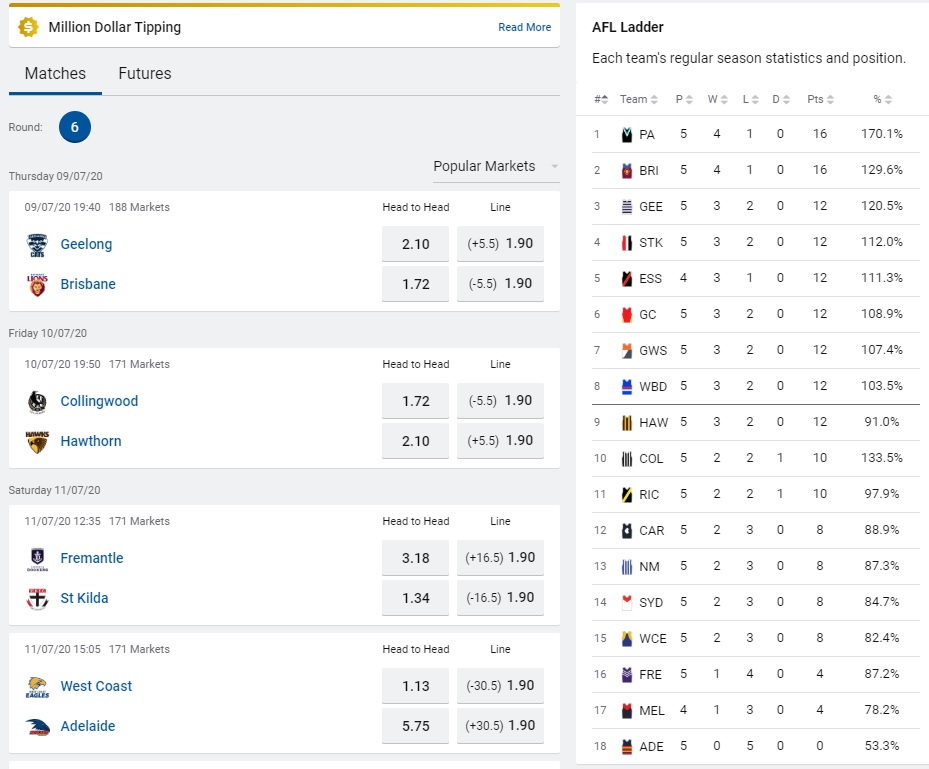This image depicts the interface of the Million Dollar Tipping platform, showcasing detailed information about upcoming matches and team statistics. On the left-hand side, there's a section titled "Matches and Futures," with "Matches" underlined in blue, indicating it's the current view. A blue circle with the number 6 is displayed, denoting Round 6.

Highlighted in blue, there's an option to "Read More," and beneath that, a list of matching fixtures scheduled for Thursday, 9th July 2020, with a total of 185 markets available. Specifics include the time 19:40 and popular market names like Geelong, Brisbane, Collingwood, Hawthorne, Fremantle, St. Kilda, West Coast, and Adelaide. A "Head to Head" column summarizes competitions, showing a sequence that spans Thursday, Friday, and intermittently through the months.

On the right-hand side, the "AFL Ladder" is presented, detailing the current standings of Australian Football League teams along with their season statistics. Teams are enumerated from 1 through 18, with each row providing comprehensive data on their performances. This well-organized layout serves viewers with a comprehensive overview of both match fixtures and team standings, aiding them in making informed tips and predictions.